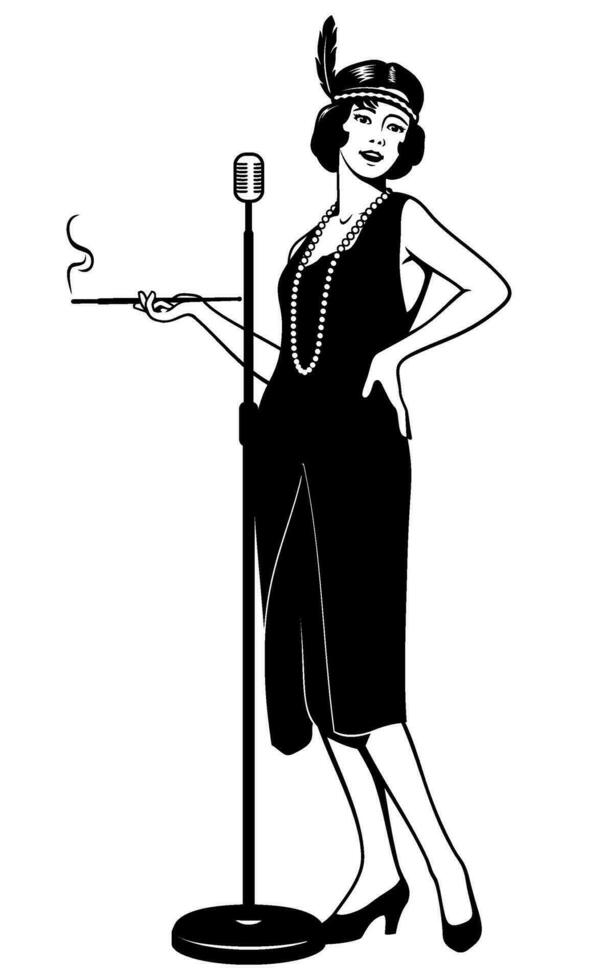This is a detailed black-and-white illustration of a young woman exuding 1920s flair, poised with a microphone stand in front of her. Her dark, chin-length hair is parted in the middle and adorned with a headband featuring a prominent feather on one side. She wears a black, sleeveless knee-length dress akin to flapper fashion, accessorized with a long string of white pearls draped elegantly around her neck. Characteristically fashionable for the era, she has on black high-heeled shoes. In her right hand, she holds a long cigarette holder emitting a wisp of smoke, while her left hand is confidently placed on her hip, adding to her striking pose. The intricate details of the image, such as the slit in the dress revealing more black fabric beneath and her swayed, stylish stance, underscore her vintage allure, evoking the atmosphere of a 1920s or 1930s performance.